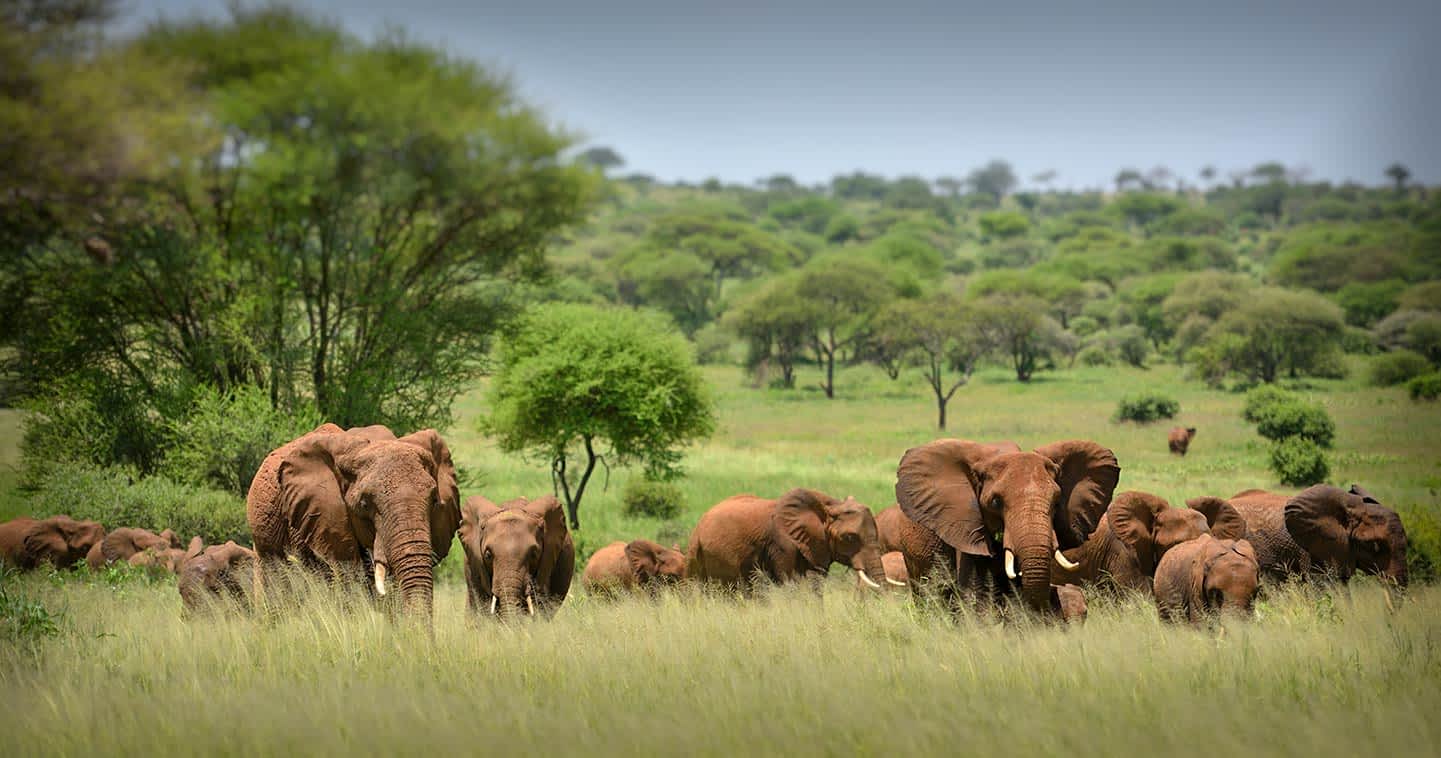This is a beautiful landscape photograph capturing a large, cohesive herd of elephants in a vibrant African setting. The group of elephants, consisting of adults, juveniles, and at least one or two babies, stands together in a clearing of tall, dry grass. The elephants' grayish-brown skin contrasts with the green, healthy trees in the background, indicative of a post-rainy season. The foreground is dominated by the high grass, adding texture to the scene, while the background features a mix of dense trees and some taller ones on the left, stretching towards a clear, grayish-blue sky. Two large elephants are prominently leading the herd, while younger ones follow closely, seemingly content and unthreatened. The detailed composition suggests a moment of foraging or perhaps a journey towards a watering spot, encapsulating the essence of their natural habitat.